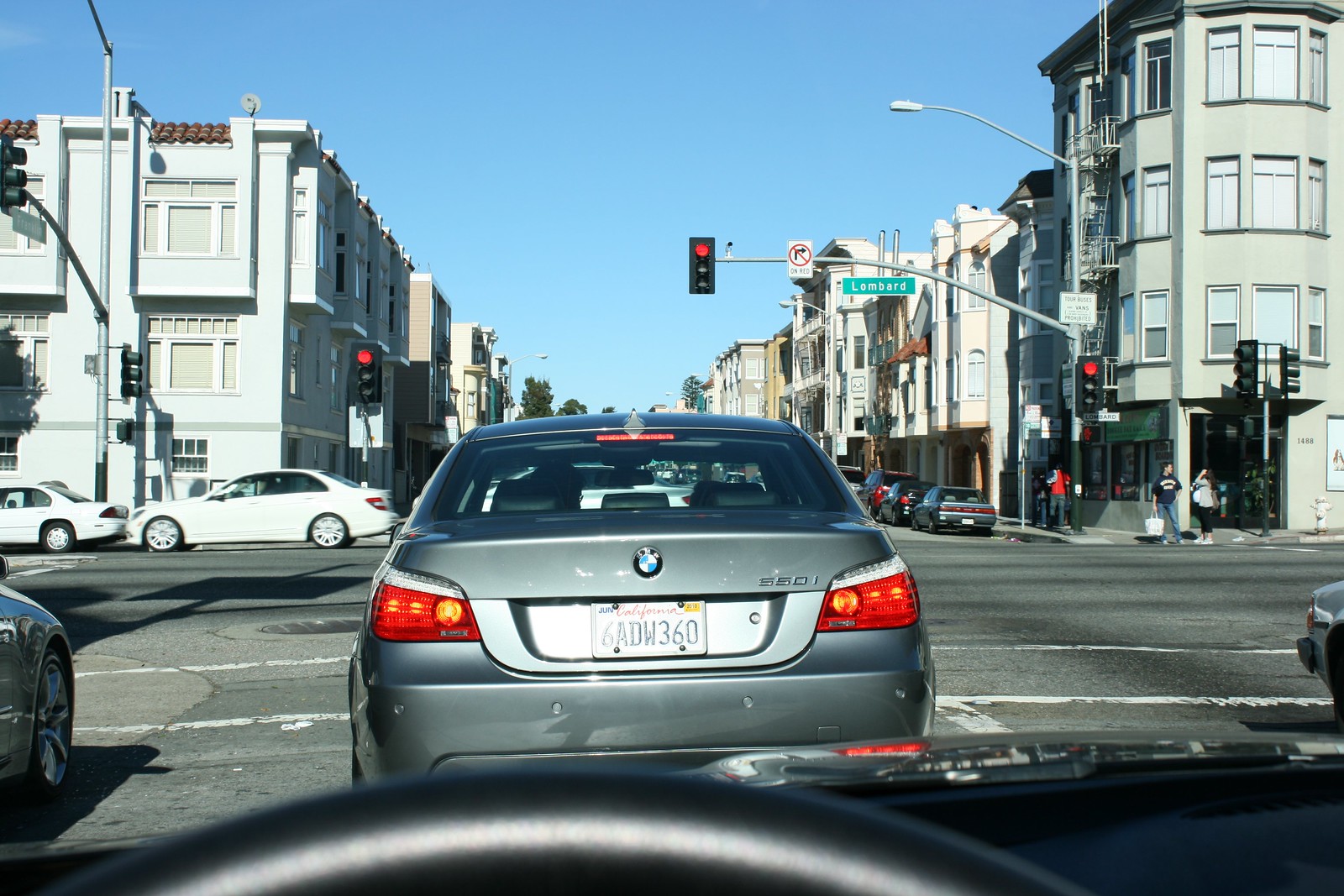This image is a horizontal photograph depicting a daytime city intersection scene under a clear, bright blue sky. From the driver's seat of a car, we see the black steering wheel at the bottom of the frame, indicating the photo is taken from inside a vehicle. Directly ahead, a light gray BMW 550i is stopped at a red traffic light, displaying a California license plate with the number 6ADW360. The intersection is identified by a green street sign labeled "Lombard." 

Flanking the street are various buildings that are two to three stories tall, combining residential spaces with ground-level stores. Along the left side of the road, two white cars are parked facing the nine o'clock direction. These details suggest an urban environment. The road appears slightly worn, with white crosswalk lines in need of some maintenance. 

On the far right corner of the intersection, several people are presumably waiting to cross the street, adding to the bustling city atmosphere.